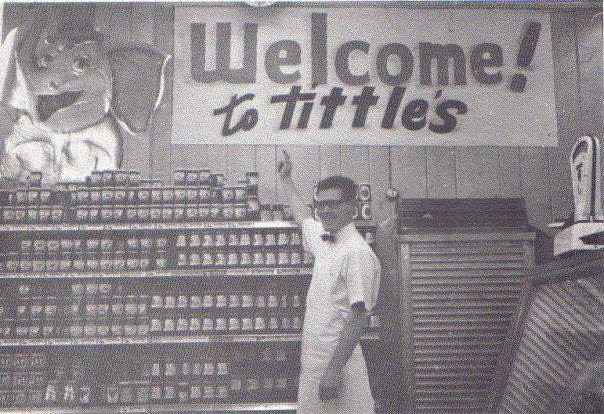A meticulously detailed, black and white photograph captures the interior of a vintage grocery store. Dominating the backdrop is a well-organized display of canned goods, neatly stacked against the back wall. In the foreground, positioned centrally, stands a man dressed in a crisp white shirt paired with a stylish black bow tie. His body is angled to the left, yet he engages the viewer with a direct gaze, his head turned slightly towards the camera. Adding a dynamic element to the scene, his right hand is raised, pointing towards a rectangular, canvas sign hanging on the back wall. The sign warmly welcomes patrons with the message, "Welcome to Tiddles." Intriguingly, the upper left section of the image features a decorative elephant figure, adding a whimsical touch to the store's quaint, yet nostalgic ambiance.